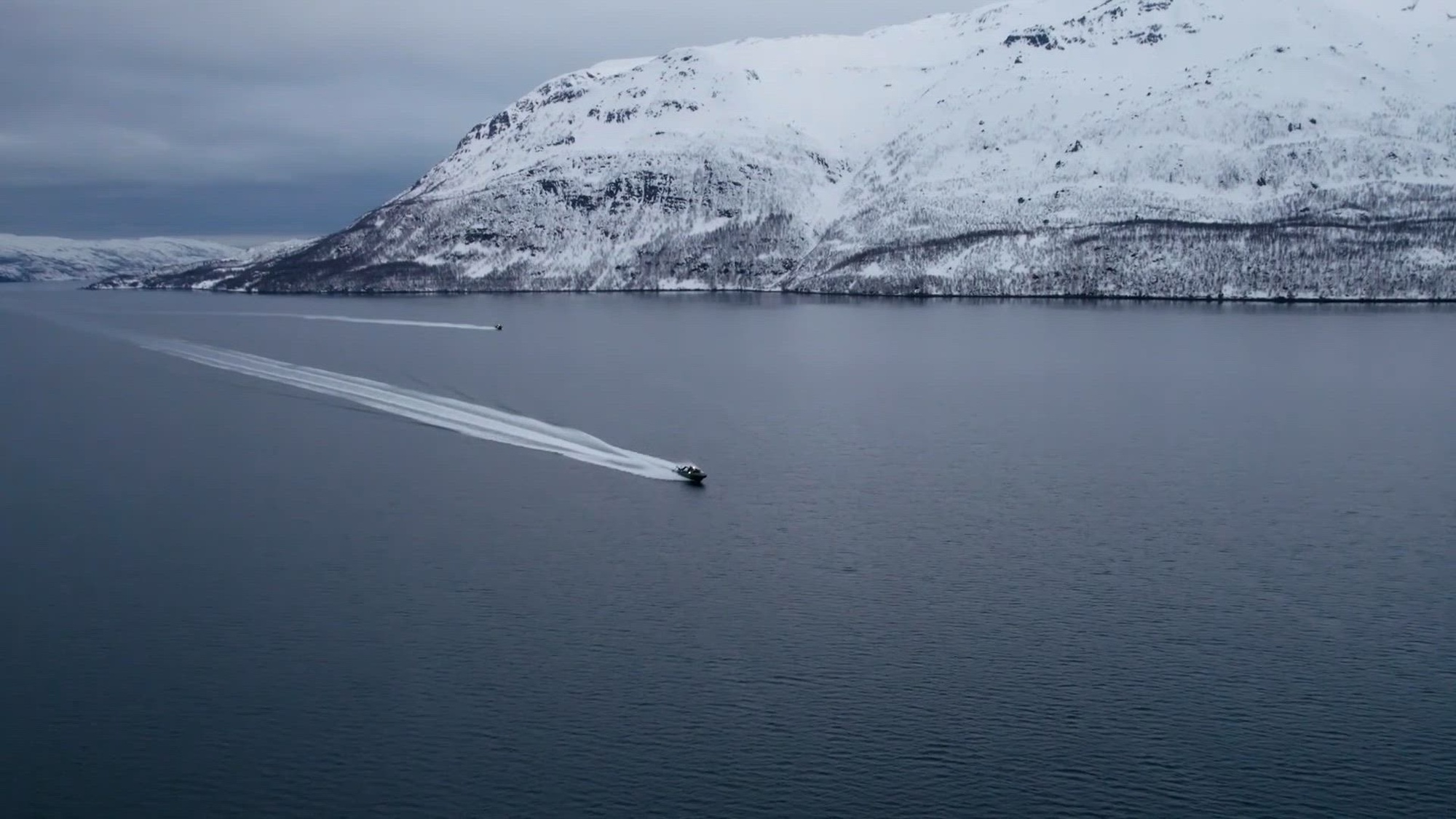This is an aerial shot, likely taken from a helicopter or drone, capturing a serene, cold setting. Central to the image is a vast body of calm water, potentially the ocean or a large lake, bordered directly by a towering, snow-covered mountain. The mountain rises abruptly from the water, with no visible shore separating the two. The scene is painted with grayish and dark bluish hues, hinting at a wintry, overcast day, though the sky is clear with some clouds. In the water, a few small boats or jet skis are moving swiftly, leaving discernible trails in their wake, especially one near the middle of the image. The tranquil expanse of water and the majestic, icy mountain frame create a breathtaking and isolated panorama.